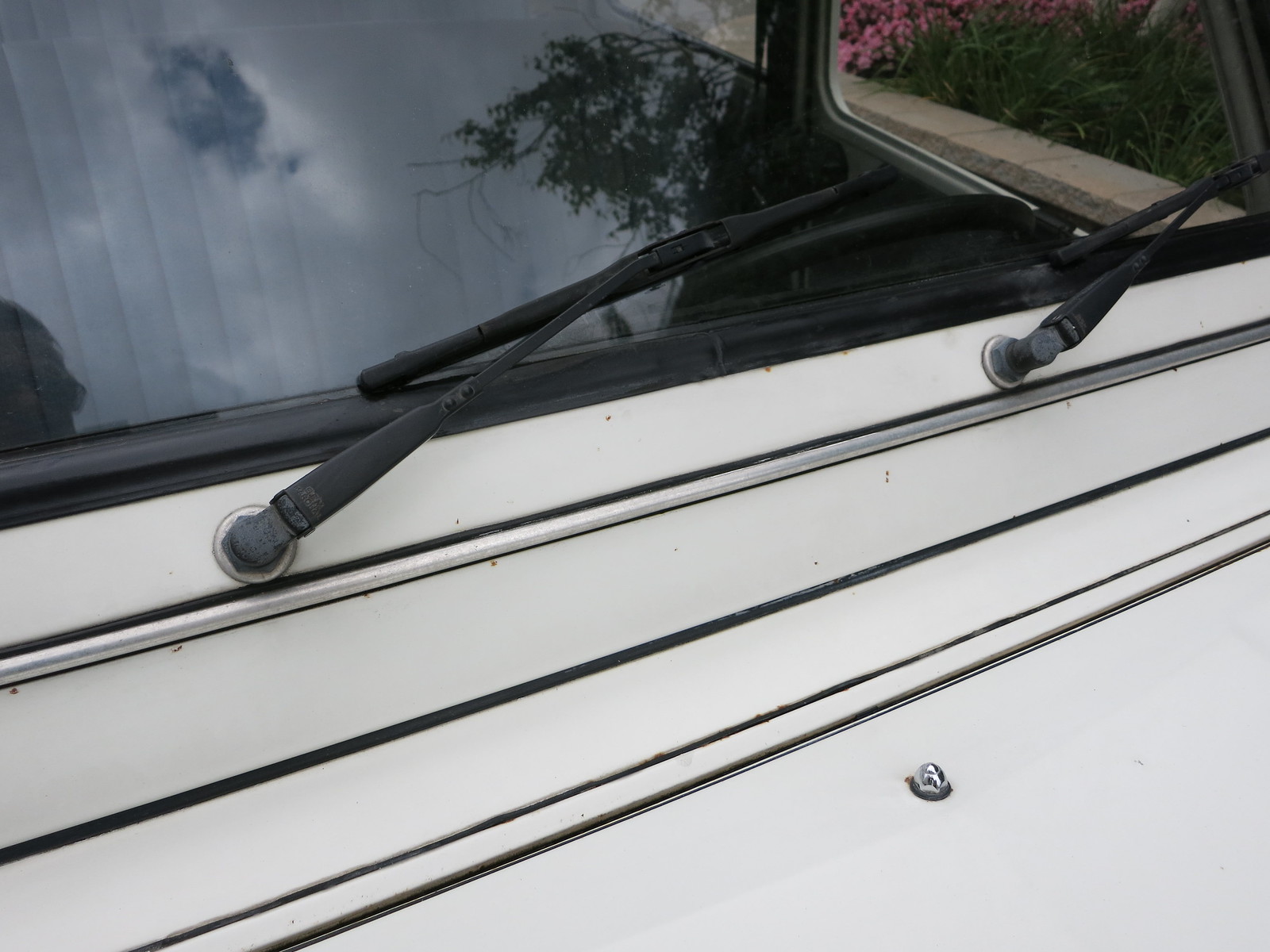This close-up photograph depicts the front section of an older vehicle, likely from the 1970s or 1980s, with a white exterior adorned with small black stripes. The image prominently features two short, black windshield wipers resting on the windshield, and the base of the wipers shows signs of rust. The surrounding black rubber seal is visible, indicating the age and wear of the vehicle. Through the slightly darkened and shadowed windshield, we can glimpse a black steering wheel and part of the interior. The driver's side window, partly in shade, reflects a dark green tree and overcast skies with a small section of blue sky peeking through. On the side of the vehicle, the black trim around the door is evident. Lastly, the front of the vehicle has visible windshield washer fluid nozzles where fluid would be dispensed.